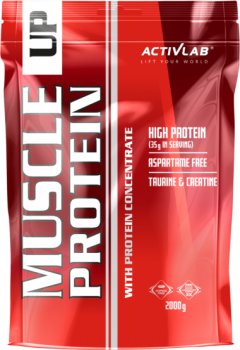The image showcases a detailed photo of a protein supplement bag, primarily in red and maroon, that appears to be resealable. The product, named "Muscle Up Protein," features prominent white lettering arranged vertically. The word "Muscle" is in a special font that resembles flexing muscles. The bag includes a vertical strip with double white lines running down the center. 

In the top right corner, it says "ACTIVLAB" with the V stylized as a checkmark, followed by the slogan "Lift Your World". The bag highlights "High Protein 35 grams per serving" and "Aspartame-Free" in white text. Beneath these, it mentions key ingredients like "Taurine," "Creatine," and "Creatinine," along with a weight indication and some seals on the bottom right that are difficult to read. The labeling emphasizes the product's protein concentrate content.